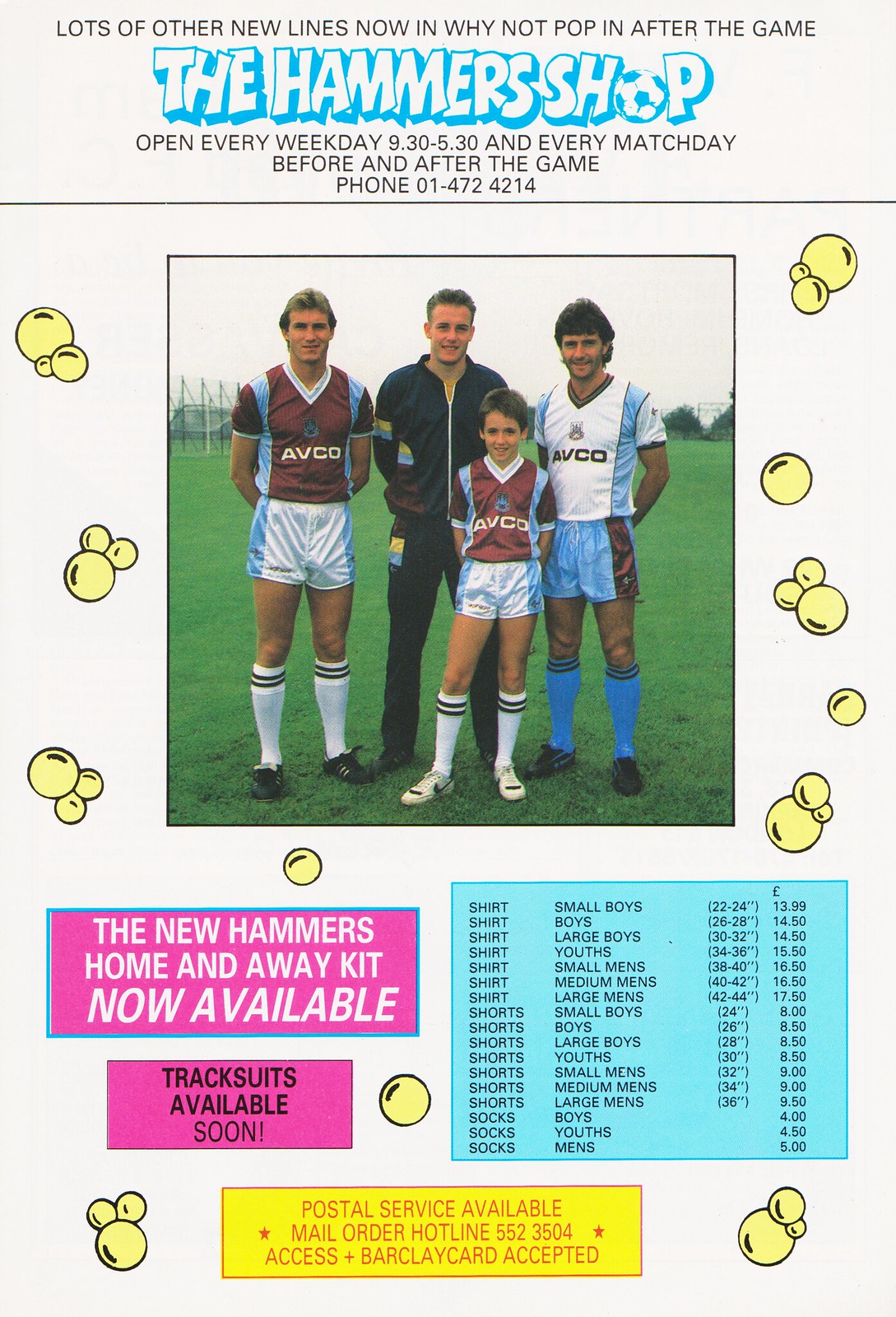The image is an advertisement from a soccer program, printed on off-white paper. At the top, it states in black font, "Lots of other new lines now in, why not pop in after the game?" Below that, in white font with a blue outline, it reads "The Hammer Shop," with the 'O' styled as a soccer ball. The shop's hours are listed as "Open every weekday, 9:30 to 5:30, and every match day, before and after the game," with a contact phone number, 014-724-214. 

The central photograph features four people standing on a soccer field: three men and one younger boy. The man in the back center is clad in a black tracksuit with sweatpants and a jacket, while the men on the right and left are wearing "Avco" jerseys—one in white and blue, the other in maroon and blue. The boy is dressed in the same outfit as the man on the left, indicating a team association.

Surrounding the image are yellow bubble drawings on a white background. Below the photograph, pink boxes convey crucial information in both white and black fonts. They announce that "The New Hammer's Home and Away Kit is now available" and that "Track suits will be available soon." Additional details include a mail order hotline, sizes ranging from small boys to adults for shirts, shorts, and socks, and payment options, including Access and Barclay cards.